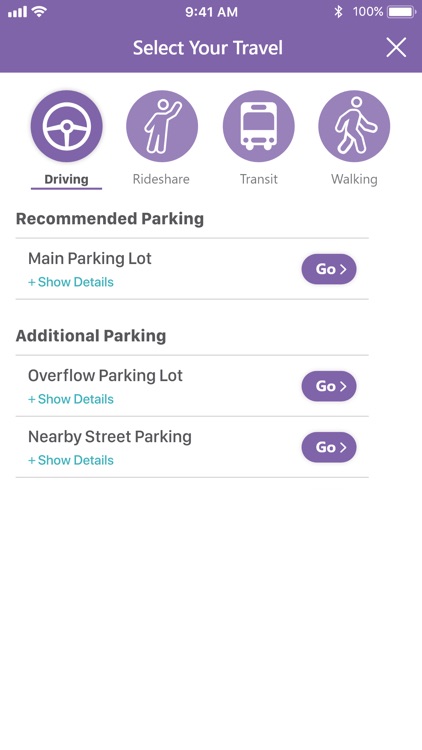A screenshot from a travel app is displayed, showcasing a user interface where you can select your mode of transportation: driving, rideshare, transit, or walking. The current selection is “Driving,” and the app provides detailed options for parking, including recommended parking spots such as the main parking lot, additional parking, overflow, and nearby street parking. The overall design features a white background with purple accents near the top and on some buttons, providing a minimalistic yet functional aesthetic. Icons are used to represent each mode of transportation: a steering wheel for driving, a crosswalk symbol for walking, and a bus for transit, enhancing the intuitive navigation of the app. The app seems to focus on helping users find the best routes and parking options based on their chosen mode of transportation.